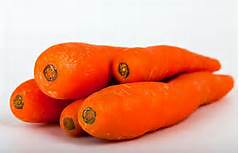This image is a detailed photograph of five bright orange carrots, arranged in a cluster. The carrots vary in size with some larger and some smaller ones. They are stacked on each other in a front-facing view, with the round, stem-removed bases pointing toward the camera, prominently displaying the tiny black circular marks typical at their bases. The tapered ends of the carrots extend outward and away from the viewer. The photo appears to be very small in dimensions, approximately 1 inch tall and 2 inches wide. The background is a grayish-white color that matches the surface upon which the carrots are resting, reinforcing the idea that the setting is likely an indoor environment.